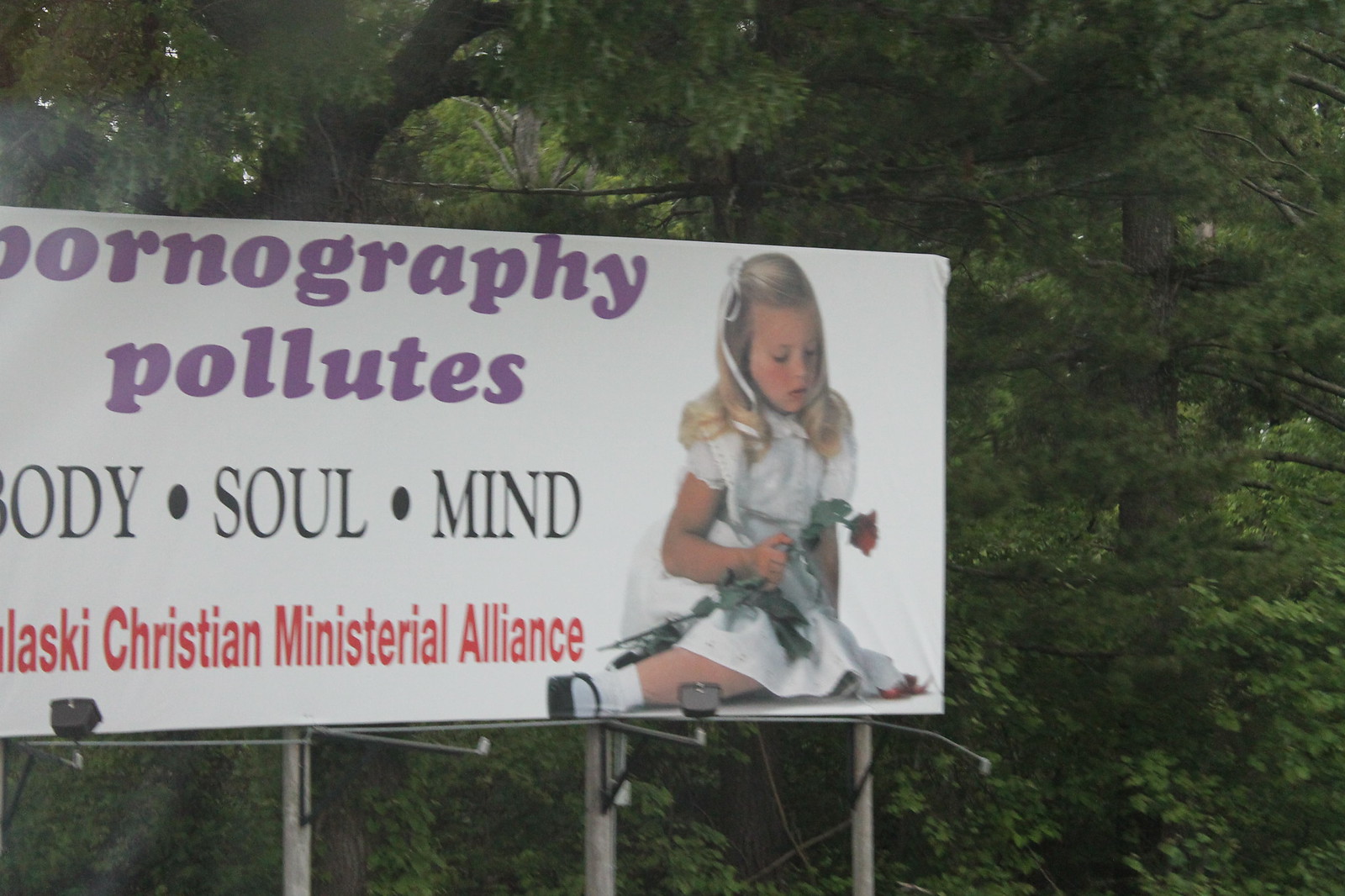This photograph captures a large billboard set against a backdrop of lush green trees with some visible brown branches. The billboard, mounted on sleek silver poles, features a white background. At the top of the billboard, a message in a purple font reads, "Pornography Pollutes." Beneath this, black text lists the effects on "Body, Soul, Mind." At the bottom of the billboard, partially obscured red text indicates the affiliation, starting with "L-A-S-K-I," followed by "Christian Ministerial Alliance."

To the right side of the billboard, there is an image of a little girl. She is dressed in a frilly white dress with a matching white ribbon tied in her blonde hair. The young Caucasian girl wears black shoes paired with white socks and is seated while holding a slightly wilted red rose. The overall composition adds a poignant contrast to the billboard message with the innocence and solemnity of the little girl's image.